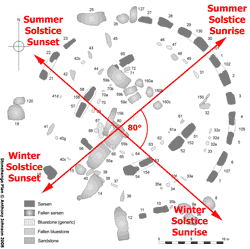This image is a detailed diagram of Stonehenge, illustrating the positions and angles of the sun during various solstices. The diagram is primarily in shades of gray and white, with a key at the bottom that is somewhat blurred and difficult to read, but attempts to differentiate various features of the Stonehenge site. In the center of the image, there is a prominent large "X" made up of two intersecting red arrows. Each arrow is tipped at all four points, representing the solstices. The upper left corner of the diagram is marked "Summer Solstice Sunset," the upper right is labeled "Summer Solstice Sunrise," the bottom right indicates "Winter Solstice Sunrise," and the bottom left shows "Winter Solstice Sunset." Additionally, the intersection angle between the arrows is marked as 80 degrees. The background includes smaller gray circles, likely representing the stones or land formations of Stonehenge, highlighting its ancient astronomical significance.